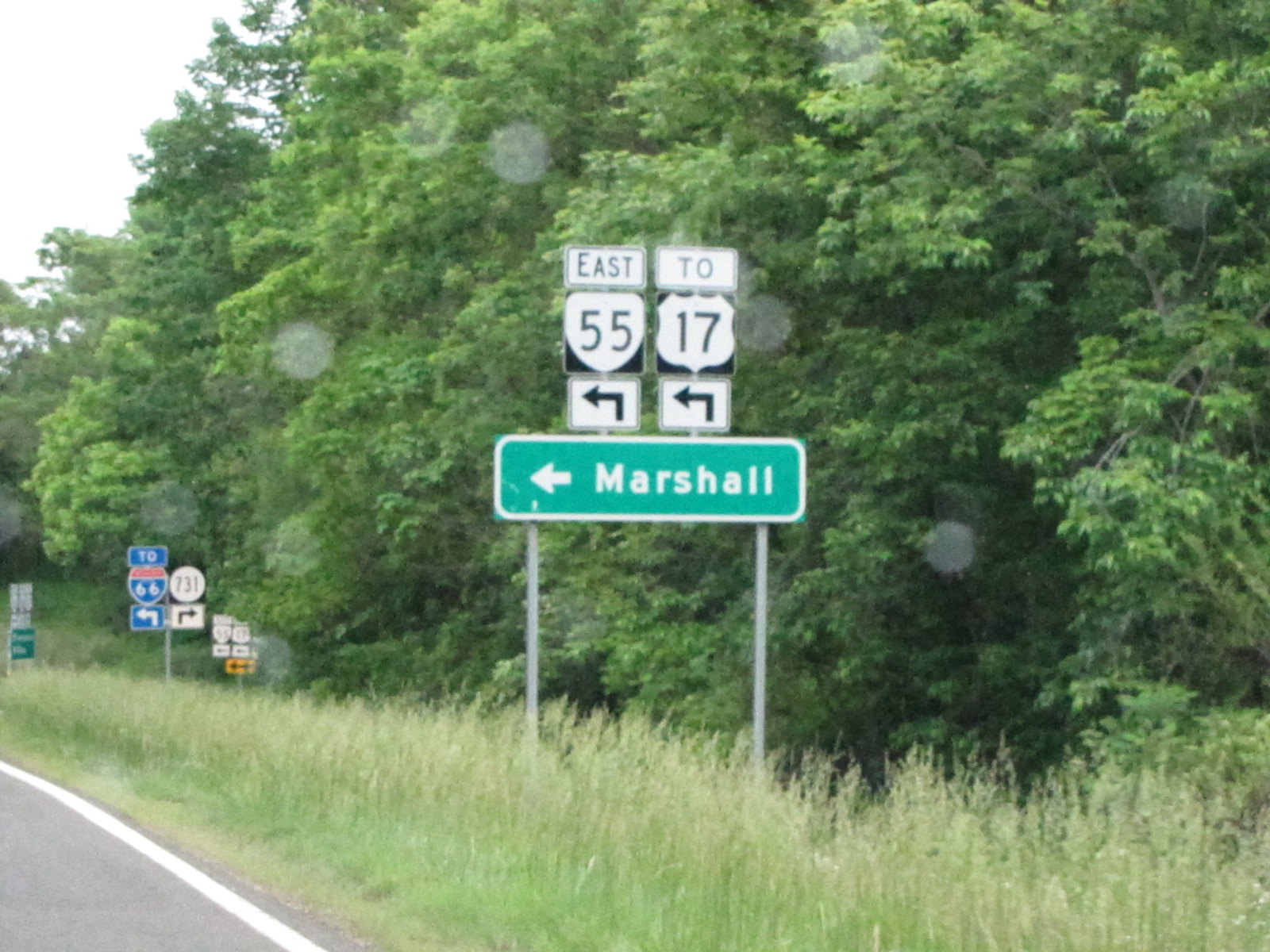The photograph captures a complex freeway junction with multiple exits directing traffic in various directions. Recognizable by the lush green trees lining the sides of the road and the tall grass, which resembles wheat strands, the image provides a scenic view. Prominently displayed is a green sign with white lettering indicating "Marshall," pointing to the left. Above this are two white signs with black numerals, designating Highway 55 and Highway 17, both directing eastbound traffic to the left. Additionally, a distinctive red, white, and blue Route 66 sign points leftward toward the historic route. Further, a white sign indicating Highway 731 directs traffic to the right. Complementing these are several other freeway signs, including a yellow T-intersection warning sign with black left and right arrows, providing essential information for navigating the intricate junction.